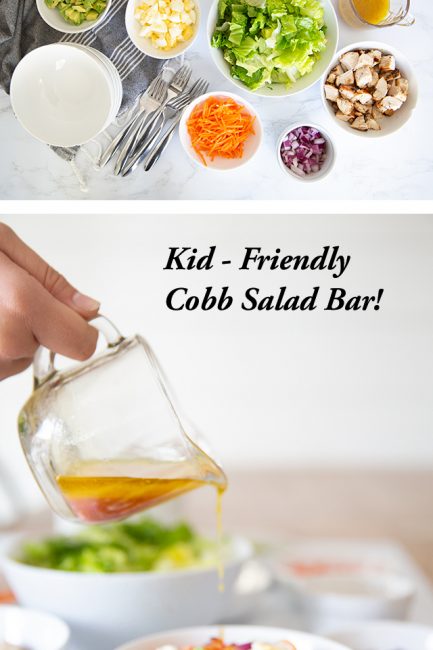This vertical image, likely sourced from a menu or advertisement, is divided into two distinct segments. The upper section prominently showcases an array of fresh salad ingredients meticulously arranged in bowls of varying sizes on a pristine white tablecloth. The ingredients include crisp lettuce, sliced mushrooms, rings of red onions, shredded carrots, green onions, and an undetermined green item. Amidst the bowls rests a small pile of salad forks, a neatly folded napkin, and a stack of white bowls, all suggesting a well-prepared salad bar setup.

The lower section features bold black lettering with the phrase "Kid-Friendly Cobb Salad Bar." This portion captures a close-up of a hand, composed of a pointer finger and thumb, pouring a brownish liquid—presumably a dressing—from a small glass measuring cup onto a fresh salad in a white bowl positioned below. The background subtly blurs out to include an assemblage of the same salad ingredients, enhancing the depth and focus on the pouring action, thus emphasizing the inviting and interactive nature of creating a custom salad from the array of available ingredients.